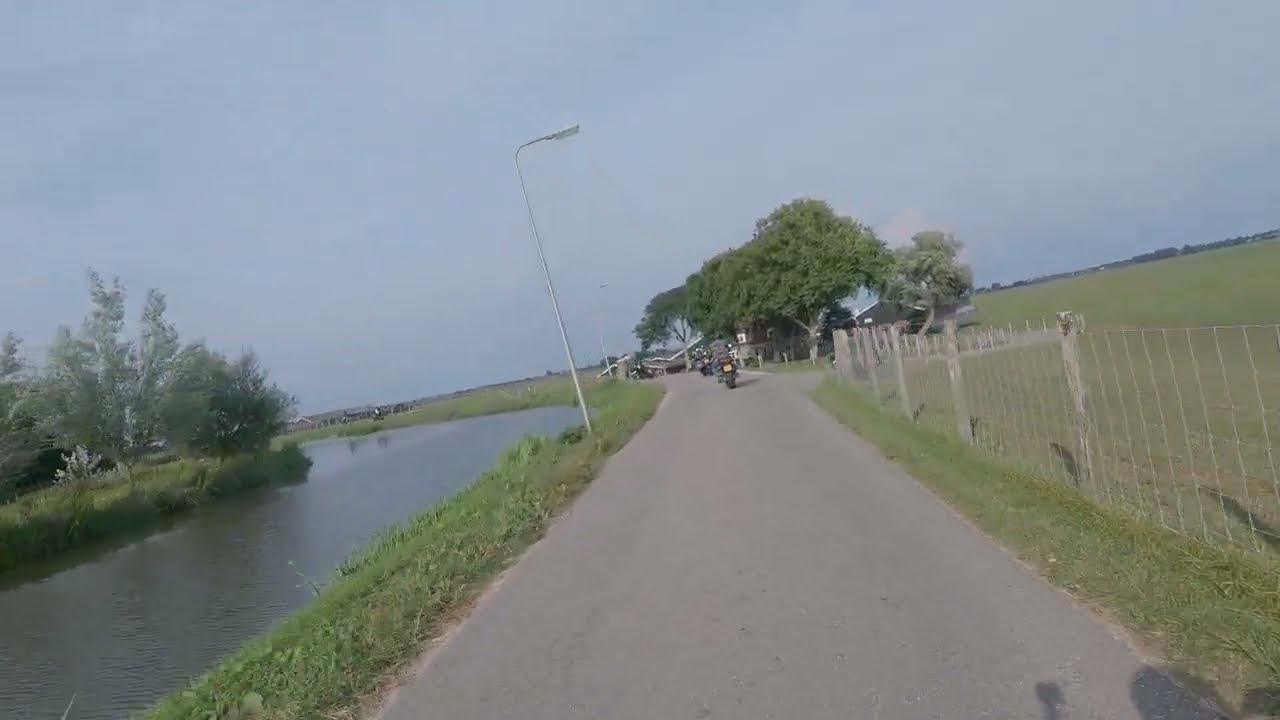The photograph depicts a serene, country road during the daytime, under a blue sky with a hint of haze giving it a nostalgic, washed-out look reminiscent of the 80s or 90s. The narrow, paved road, devoid of lane markings, snakes from the foreground towards the center before curving to the left and disappearing from view. Dominating the left side of this road is a silver metal streetlight, positioned adjacent to a calm river or canal. This water body is bordered by a patch of grass leading up to it.

Further enhancing the bucolic charm, a wire fence runs along the right side of the road, separating it from an expansive green field. As the road stretches out, a motorcyclist (or possibly two) can be observed riding towards the curve. In the central distance, just before the road bends, clusters of trees and a few houses emerge, suggesting a sparsely populated, tranquil area.

The entire scene is framed as if taken from a first-person perspective, with a faint shadow at the bottom right hinting at the photographer's presence. The overall composition, including the mix of natural greenery, quiet waterside, and minimal human activity, evokes a peaceful, park-like ambiance.